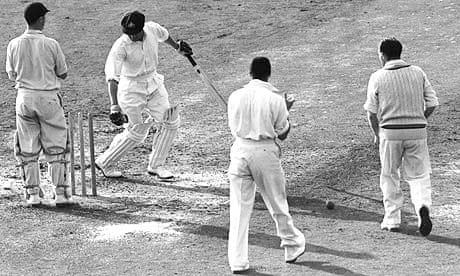This black-and-white landscape photograph appears to capture a historical game of cricket. The image showcases four men dressed in traditional cricket attire, which includes white shirts, pants, and mostly white shoes. Predominantly, they are all wearing hats, with the man on the far right distinguishing himself with a white sweater vest. The scene is set in a dirt field, likely from a bygone era, given the monochrome tones. On the left-hand side, one man is positioned behind the three sticks, commonly known as the stumps or wickets in cricket. In front of these stumps stands another player, who is equipped with a bat and donning knee pads and a dark hat. To his right, two more men are walking in the direction of the batter, and a cricket ball is visible on the ground between them. The photograph captures a moment of preparation or pause in a cricket match, emphasizing the distinctive elements of the game and the era it represents.